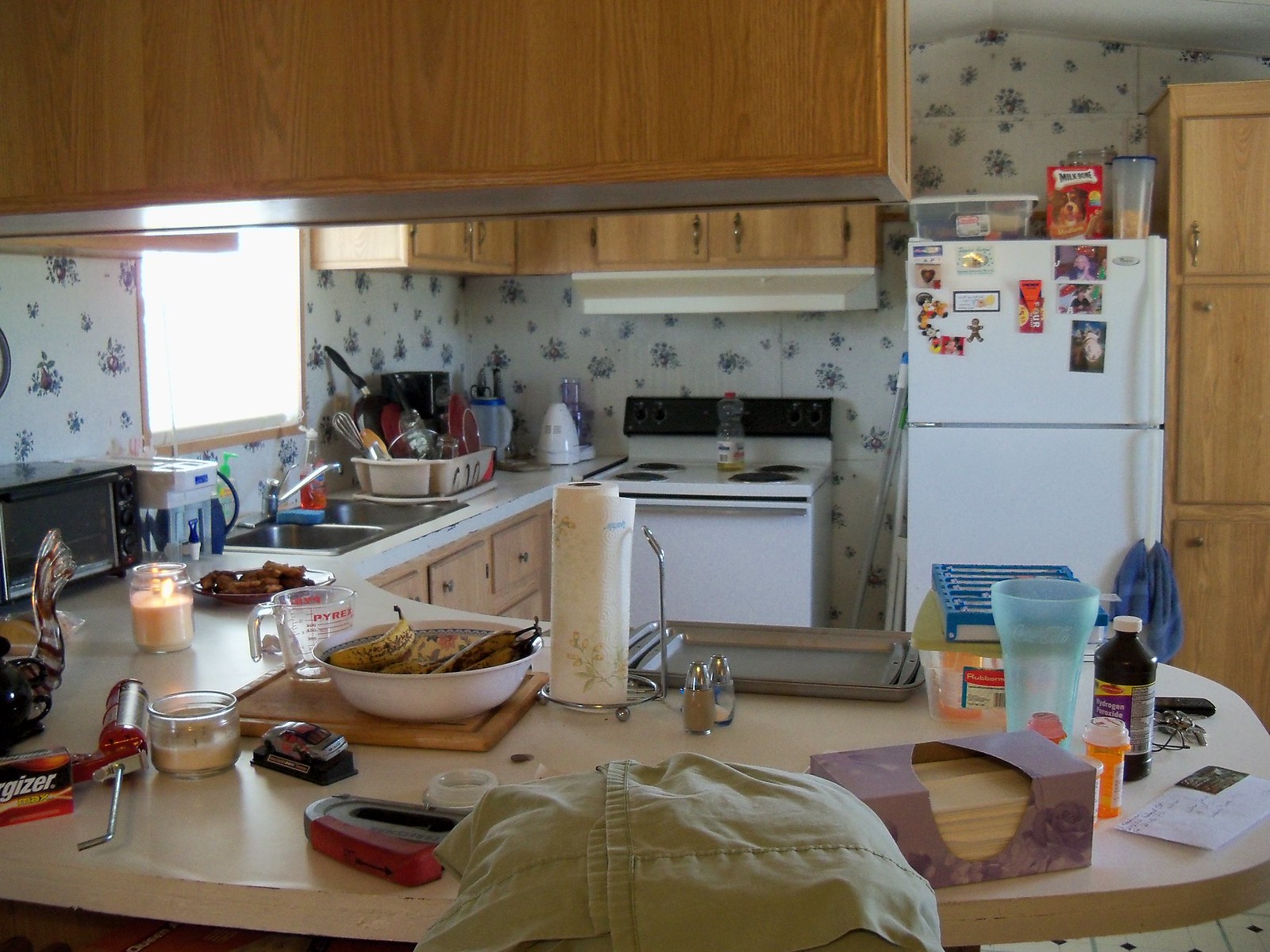This photograph captures a cozy, traditionally styled kitchen, typical of an apartment setup. The space features an older wire burner range and oven, positioned under a slightly mismatched, overextended vent hood. The oven is a vintage model, lacking a window for interior viewing. To the right stands an older style refrigerator, adorned with magnets and topped with a box of Milk-Bone dog treats.

Dominating the upper half of the kitchen are wooden cabinets that extend from above the stove, curving around a window on the left, and continuing to form a perimeter around a countertop that doubles as a bar area. This bar surface is cluttered with everyday items: napkins, cups, a plastic tub, a bottle of iodine, several medicine bottles, salt and pepper shakers, a set of sheet pans, and a wooden cutting board, which holds a bowl of slightly overripe bananas. The bar also hosts a lit candle, a caulking gun, a pack of Energizer batteries, and a compact toaster oven.

The sink area is neatly organized with various soaps and a sponge but is free of dirty dishes. To the right of the sink, a drying rack holds utensils and a pan, while water jugs and a small electric kettle are placed nearby. Overall, the kitchen exudes a practical, lived-in charm, with its eclectic mix of modern conveniences and vintage appliances.